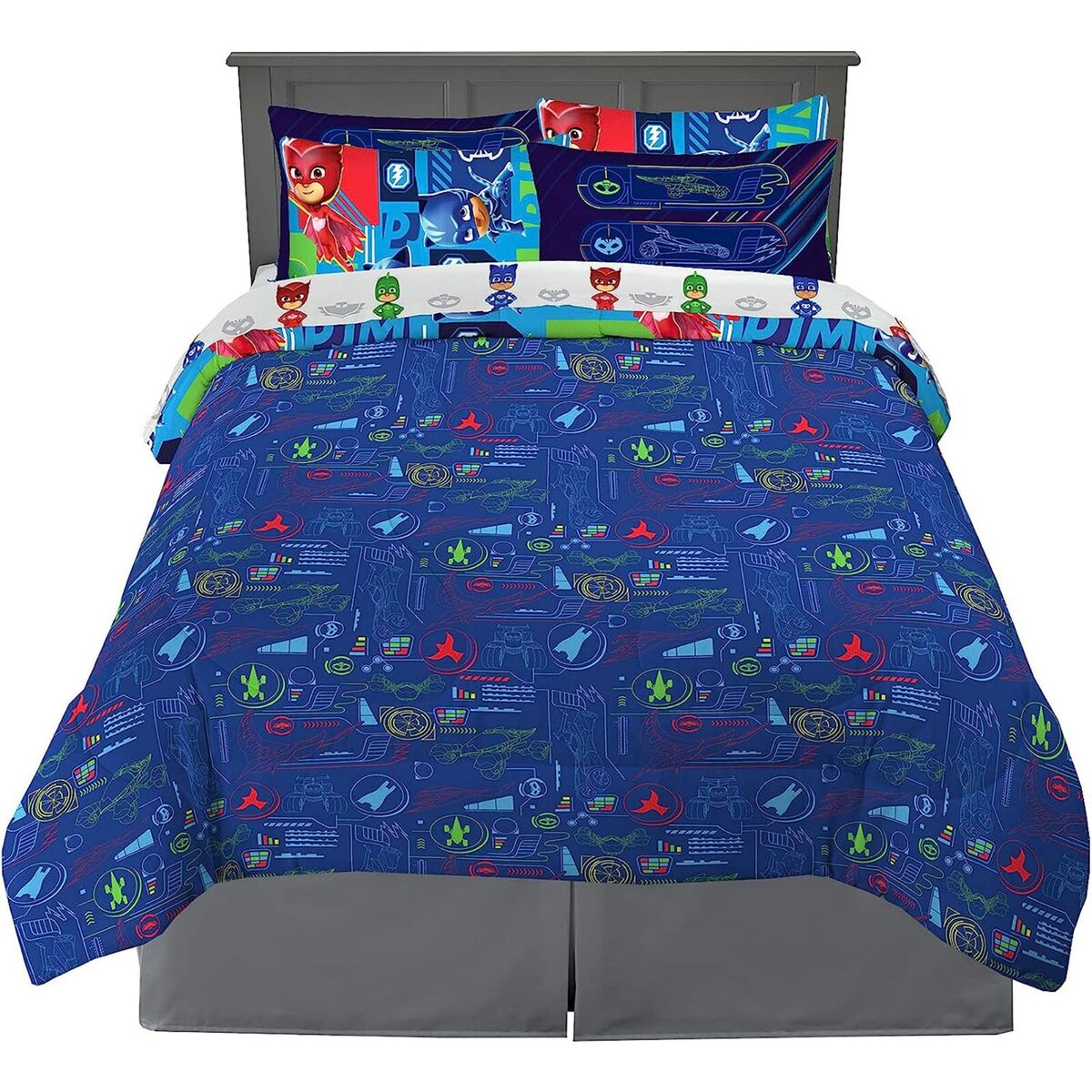The image depicts a child's bed, showcasing a combination of playful design and vibrant colors. The main body of the bed, including the headboard, is a charcoal gray color, likely made of wood. At the forefront, a dark green bed skirt suggests the presence of a box spring. Spread across the bed is a blue-colored blanket rich with kid-friendly designs like eagles, spaceships, and other space-themed icons in red, green, and blue. Nestled near the headrest are four pillows; two of them feature cartoon-like superhero characters dressed in red and blue costumes, while the other two have blue pillowcases adorned with various space vehicle illustrations. The superheroes on the pillows exhibit light, pale skin tones underneath their colorful masks and uniforms. The top part of the blanket is folded over, revealing a white underside, adding a crisp contrast to the bed's whimsical theme.